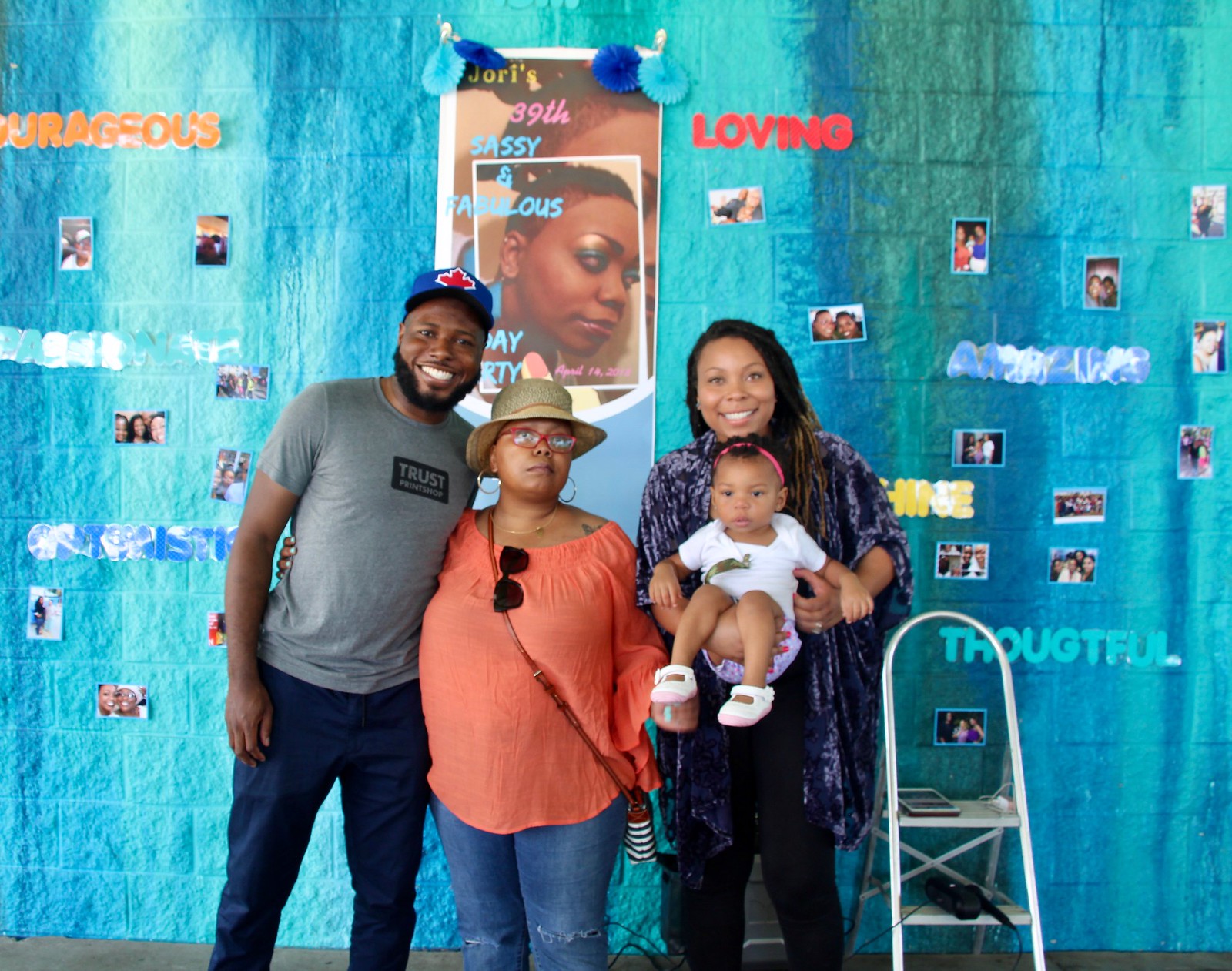This vibrant photograph captures a joyous black family of four, beautifully posed and huddled together against a turquoise, brick-patterned wall adorned with an array of photographs. These photos—likely of family and friends—are interspersed with words in various colors and Sans Serif fonts, such as "Thoughtful" in light blue, "Loving" in red, and "Courageous" in orange. Additionally, a large blue banner announces "Jory's 39th Sassy and Fabulous Happy Birthday," accompanied by an image of a woman.

On the left stands a younger black man with a warm smile, wearing a gray t-shirt reading "Trust Print Shop" in black and gray, navy-colored jeans, and a blue hat featuring a red maple leaf. He sports a black beard and has his arm around a shorter, fuller-figured black woman dressed in an orange top, ripped blue jeans, a straw hat, and red glasses. Beside her is a younger black woman wearing a long, patterned purple overcoat and black jeans, holding a young girl dressed in a white shirt, purple shorts, and white shoes. Their genuine smiles and close embrace create a heartwarming and celebratory family scene.